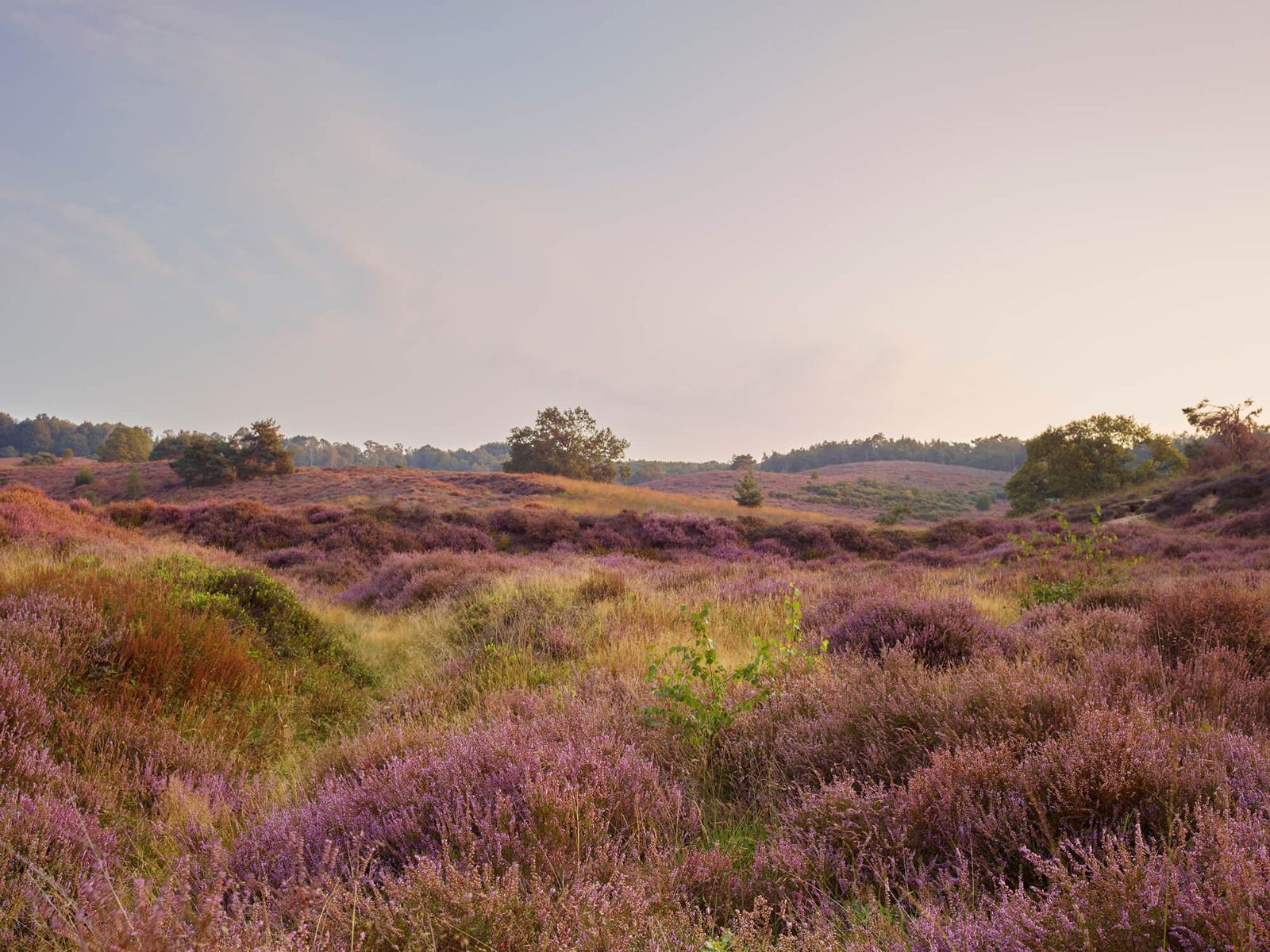The image captures an expansive, slightly hilly landscape brimming with nature's beauty. The sky is a pale blue, transitioning to a delicate yellow hue on the right, adorned with light, wispy clouds. The rolling fields are awash with dusky purple and pink flowers, resembling heather, interspersed with vibrant green grasses and sparse patches of brown. Scattered throughout the hills are green branches with small leaves and occasional bushes. As the land stretches endlessly, it seamlessly meets a distant tree line punctuated by tall, lush green trees. The overall ambiance is tranquil and picturesque, suggesting an infinite expanse of serene prairie under an expansive sky.